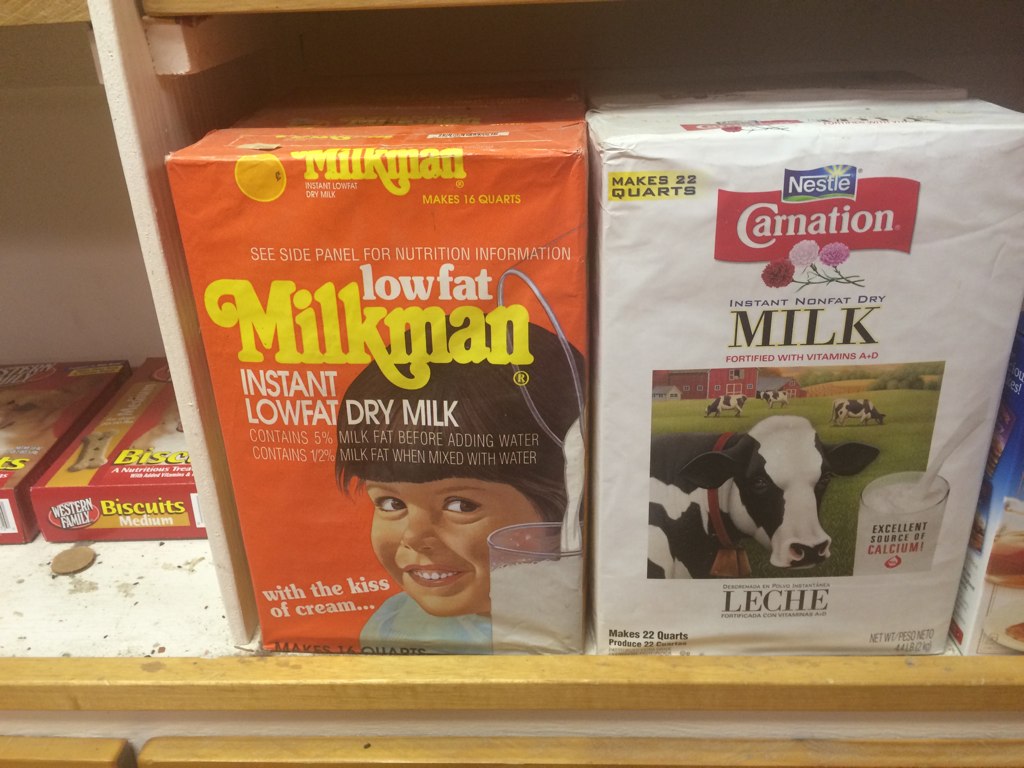This photo depicts a shelf inside what appears to be a brown wooden cabinet. The cabinet door is open, revealing a white, somewhat dirty shelving unit with a white wooden divider separating it into two sections. There's also brown wood trim on the front of the shelf. On the left side of the shelf sits an orange box of Milkman instant low-fat dry milk, which features the slogan "with a kiss of cream" and an illustration of a smiling child with brown hair and brown eyes, glancing sideways while holding a glass of milk. Milk is shown being poured from a pitcher into a glass on the box. To the right of this box is a white carton of Nestle Carnation instant nonfat dry milk fortified with vitamins A and D, boasting that it makes 22 quarts and is an excellent source of calcium. The box displays an image of a black and white cow with a brown belt around her neck and additional cows in the background grazing in front of a red barn. Additionally, there are two boxes of Western Family medium-sized dog biscuits lying down on the far left side of the shelf, and a small penny can be spotted near them.